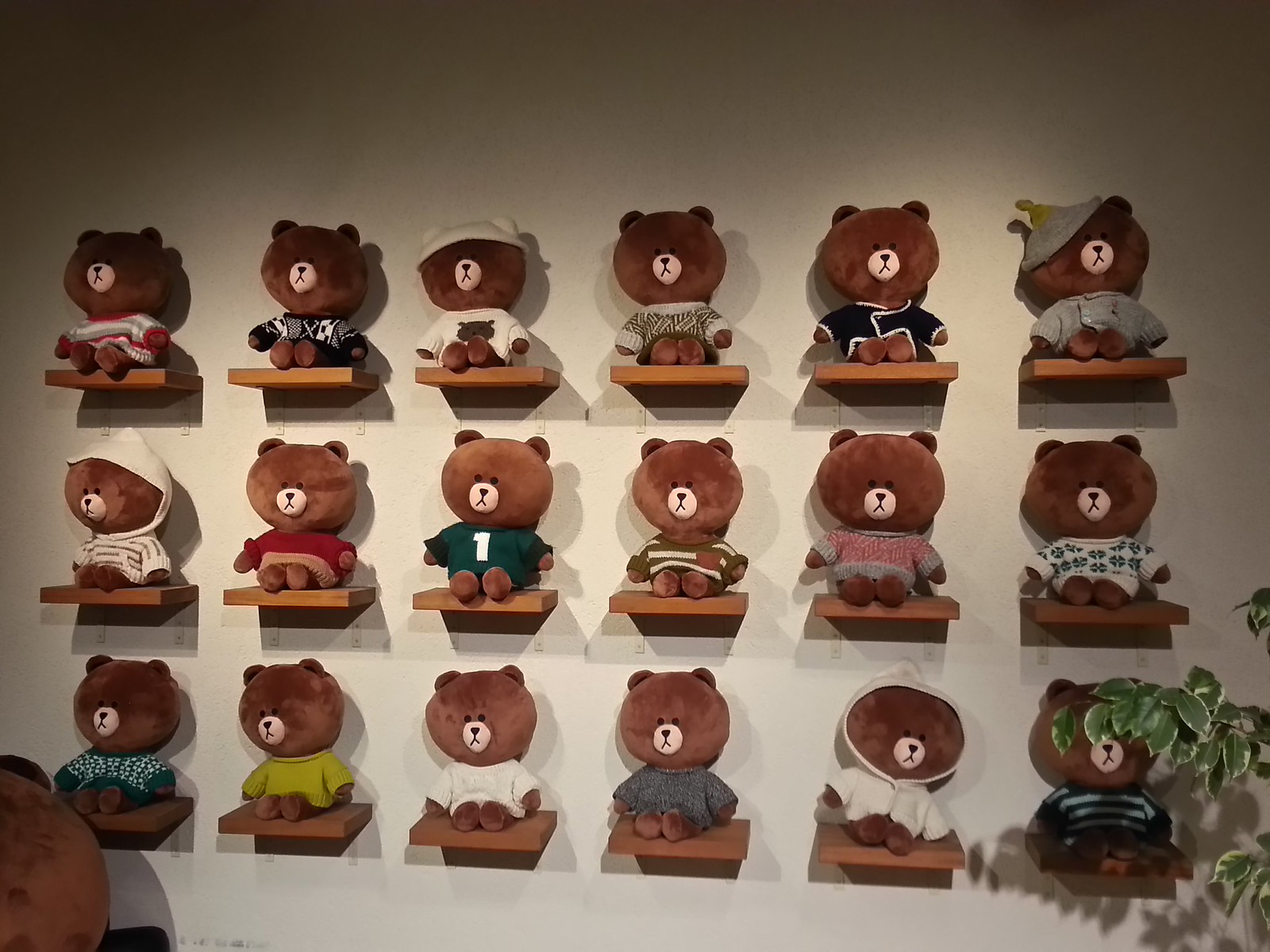This indoor photograph captures a neatly arranged display of 18 identical brown teddy bears seated on three rows of six small, square wooden shelves mounted on a light gray, white, and subtly gradient wall. The teddy bears, all identical in their physical characteristics with round fuzzy heads, dot eyes, Y-shaped mouths, and white snouts, are differentiated by their unique outfits. Some are wearing distinct shirts, jerseys, or sweater dresses in colors such as red, green, white, yellow, black, and grey, while others sport hats or hoods. Notably, one teddy bear on the second row wears a blue shirt with the number one. In the bottom right corner, green leaves from a plant slightly obscure one of the bears, adding a touch of natural element to the meticulous arrangement. The background is simple, allowing the whimsical variety of the teddy bears' attire to stand out prominently.